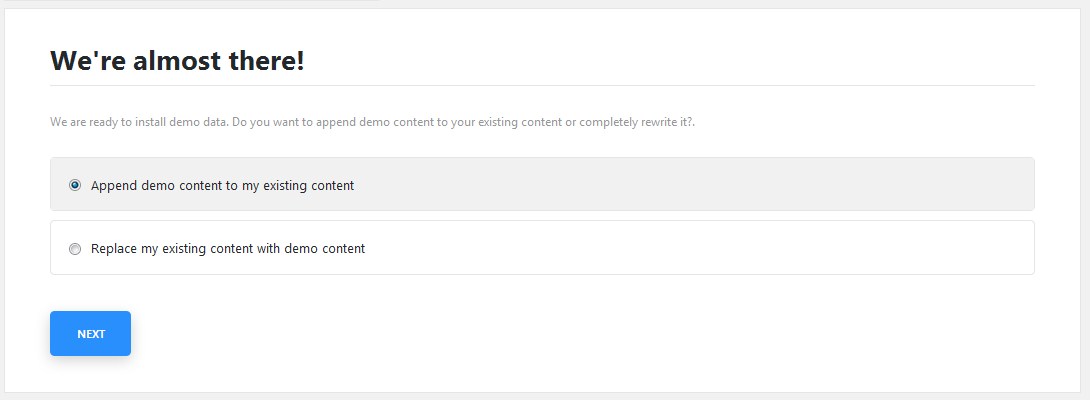The screenshot showcases a minimalistic user interface for a web-based application, possibly a content management system like WordPress. The main area features a white background with bold, black text that reads, "We're almost there!" A thin beige line underneath adds subtle contrast, accompanied by smaller black text that states, "We're ready to install demo data. Do you want to append demo content to your existing content or completely rewrite it?"

Two options are presented below this message, each with distinct styling. The first option is selected and highlighted with a yellow background and a thin border, labeled "Append demo content to my existing content," and is denoted by a filled radio button to its left. The second option, unselected and displayed on a white background with a similar thin border, reads "Replace my existing content with demo content" and features a blank radio button.

At the bottom of the interface, a solid blue button stands out with the word "NEXT" prominently displayed in capitalized white text. The entire layout suggests this is a crucial final step in configuring how demo content is integrated into a website, hinting at a blogging or web management platform.